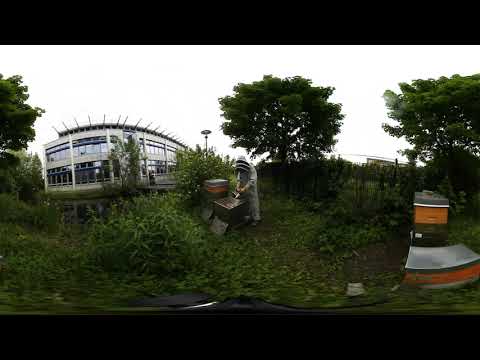The photograph captures an outdoor setting with a cloudy sky, featuring a large, white industrial building with many windows and distinctive spiky rooftops in the background. In the center of the image stands a person in a white or gray beekeeper's outfit, suggesting they are engaged in beekeeping activities, possibly fumigating or tending to the hives. Surrounding the beekeeper are several beehive boxes, identifiable by their orange and gray coloring. The scene is lush with greenery, including numerous green trees and plants, creating a natural environment around the structured beehive setup. The overall composition emphasizes the beekeeper and the hives as central elements, framed by the greenery and the imposing building in the distance.